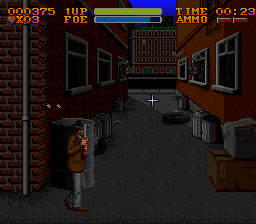The image is a detailed still from a dark, gritty computer game set in an alleyway between two buildings. On the left side of the alley, there's a man wearing blue jeans, a brown jacket, and possibly a hat tipped low over his face. He stands in the shadows next to a red brick wall with a grey gutter that extends from top to bottom. Behind him, the maroon building has two high windows, and near his feet are trash cans and large containers.

The alleyway itself is dimly lit, with the ground appearing to be dark grey, potentially asphalt or cement. On the right side of the alley, there's a red building featuring three white-rimmed windows; the middle window has a person leaning out. Below, there are more trash cans, a dumpster, and a large wooden box topped with a square stone. Among the assorted debris on this side is a single car tire lying on the ground.

In the middle of the alley, there is a prominent white cross that likely serves as the game's cursor. Across the top of the screen, various stats are displayed in an old school font: numeric codes, a green bar labeled "IVP" for the player, a blue bar for the foe, a time counter at 00:23, and an ammo counter with red indicators. The letters transition in color from yellow to red as they extend downward, contributing to the game's intense atmosphere.